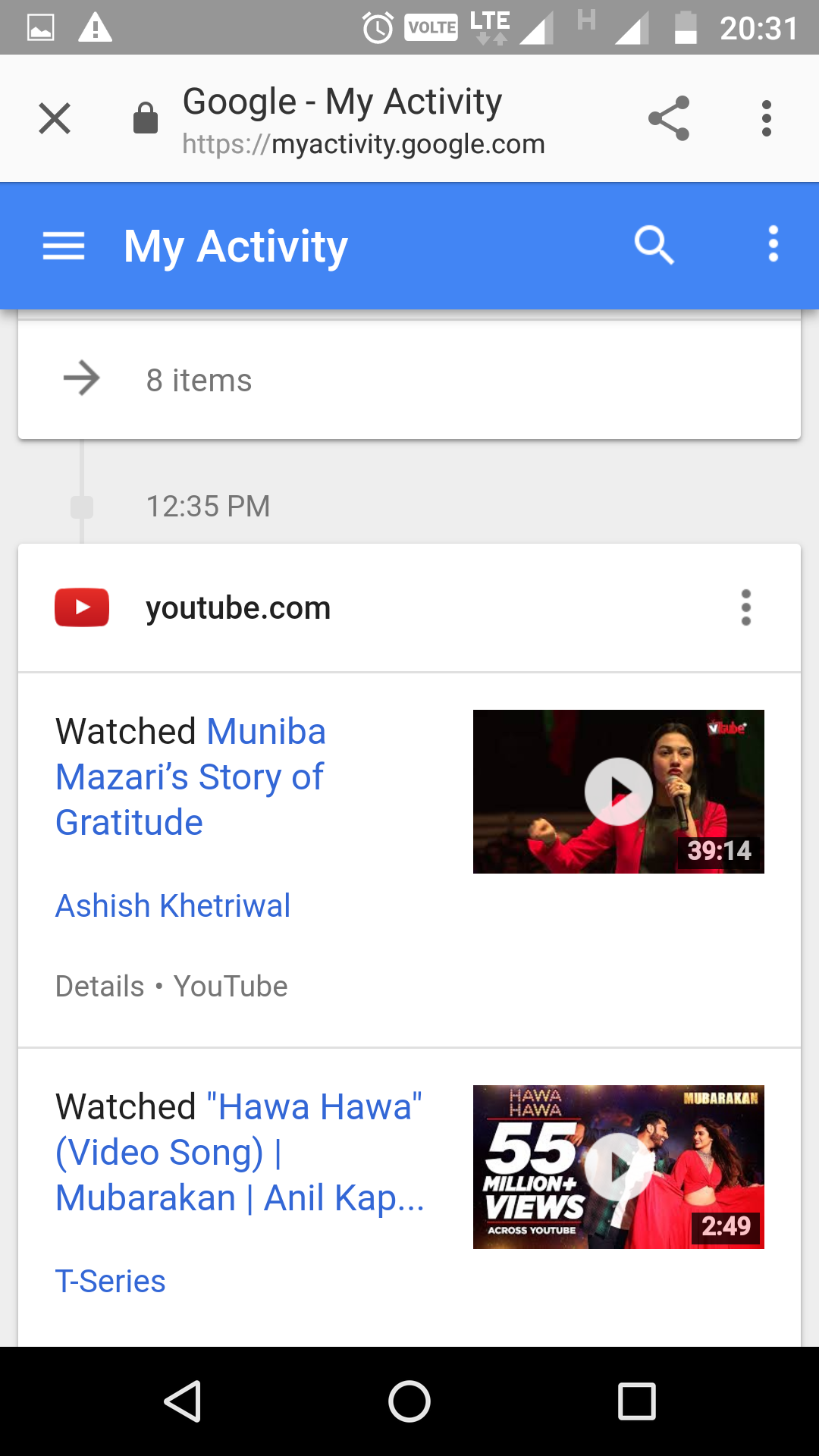Screenshot of a cell phone displaying web activity on Google’s "My Activity" page. The browser interface indicates the URL as https://myactivity.google.com, with a visible 'X' icon on the left for navigation. The device's clock reads 20:31, and multiple clickable icons are present at the top of the screen. A prominent blue rectangle is labeled "My Activity," featuring a three-bar menu icon on the left, a magnifying glass on the right, and vertical ellipsis indicating additional options. Below it, an arrow icon points right with the label "8 items." Further down, a YouTube icon alongside "youtube.com" is displayed, accompanied by a vertical ellipsis for more options. Two YouTube video entries are listed: the first titled "Watched Muniba Mazari's story of gratitude" by Ayesh Khatral, and the second titled "Watched Hawa Hawa video song," each showing the video thumbnail on the right and description on the left.